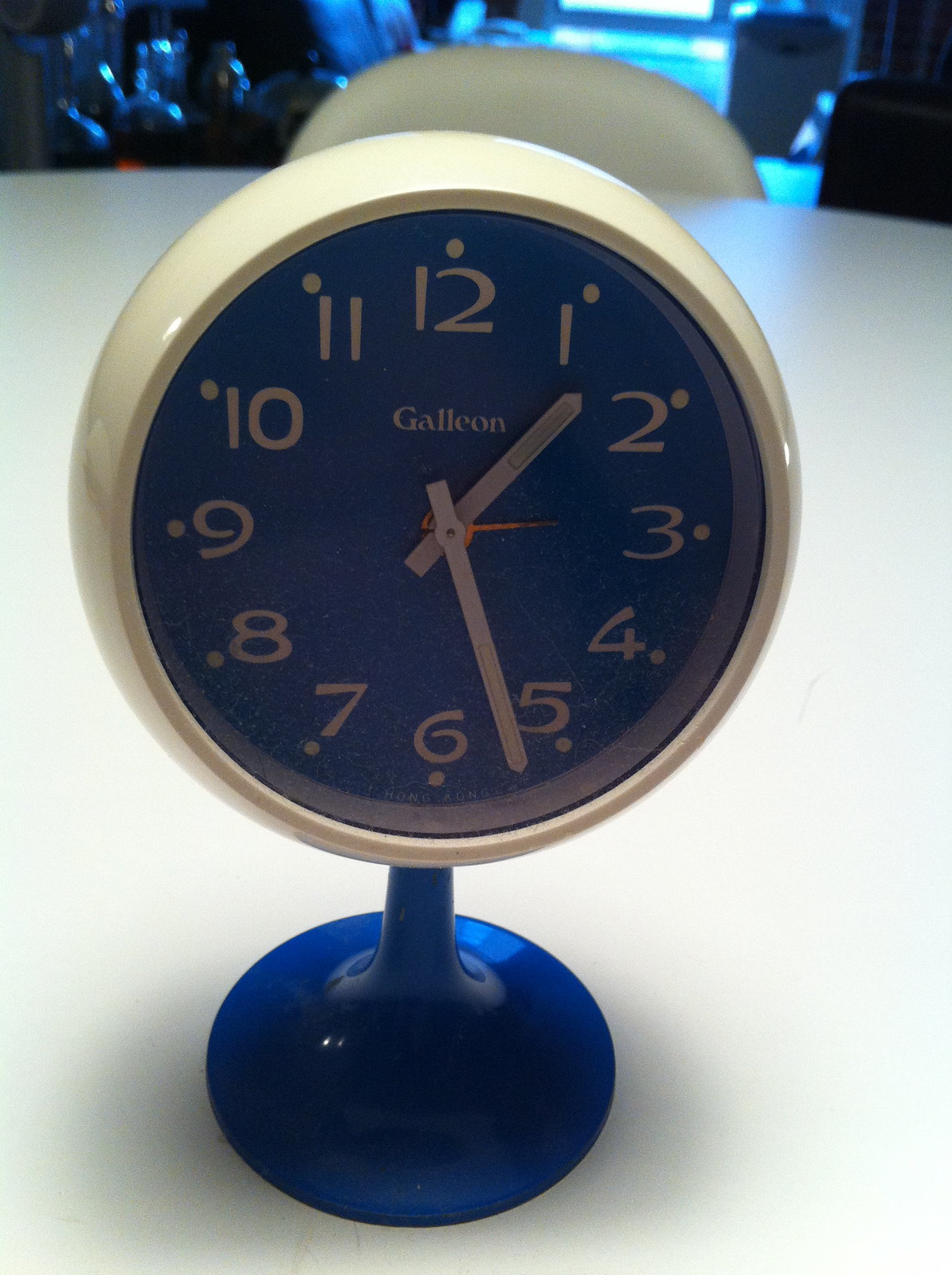A close-up photograph of a uniquely designed clock. The clock's face is vividly blue and encircled by a pristine white border. Its round shape houses numerals in crisp white font, each accentuated by a small circle above. Prominently positioned beneath the 12, the brand name "GALILEO" is emblazoned in a neat, capitalized format. The clock features three distinct hands: a short orange second hand accompanies the traditional hour and minute hands. The base of the clock, a fascinating blend of purplish hues around the edges and a dark blue center, appears to be crafted from glass, giving it a translucent quality. A sturdy stem rises from the base, seamlessly supporting the clock's face, merging function with an eye-catching aesthetic.